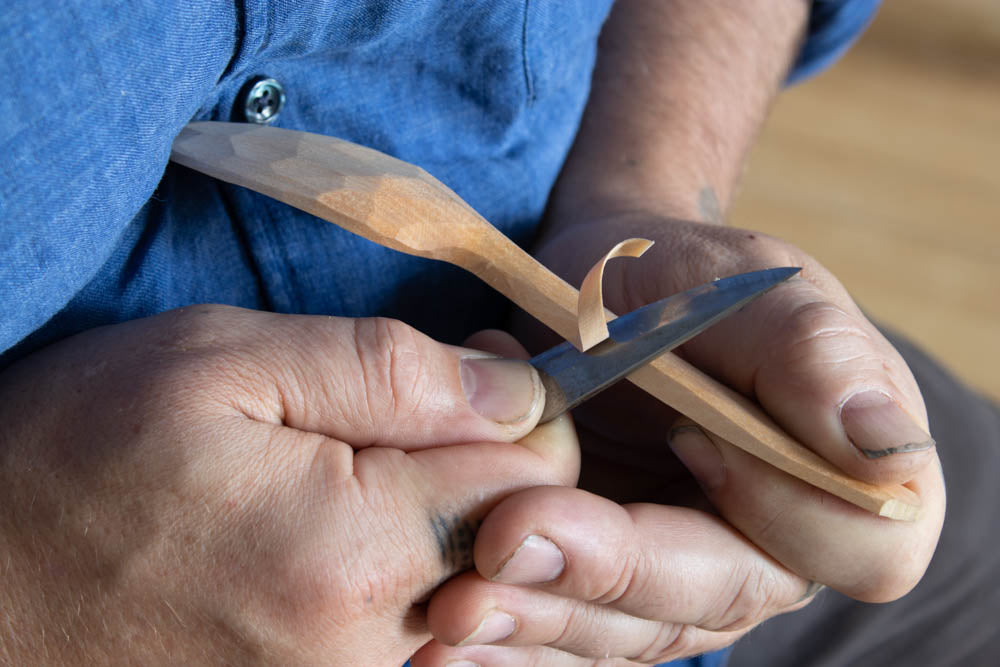The image features a close-up view of an older individual's lap, focusing on the hands as they intricately carve a wooden utensil, likely a spoon. The person is wearing a blue button-up shirt and medium-grey pants, with the utensil braced against their body. Both hands, which exhibit signs of manual labor with dirt under the fingernails, are engaged in the activity. The right hand, which appears to have a dirty thumbnail, holds a knife with the thumb on top for guidance and the pointer finger bent at a 90-degree angle at the second knuckle. The left hand grasps the wooden utensil, securing it as a small peel of wood curls away from the knife’s blade, a testament to the carving process. The hands and the knife are centrally positioned within the image, emphasizing the meticulous craftsmanship in the act of shaping the utensil.